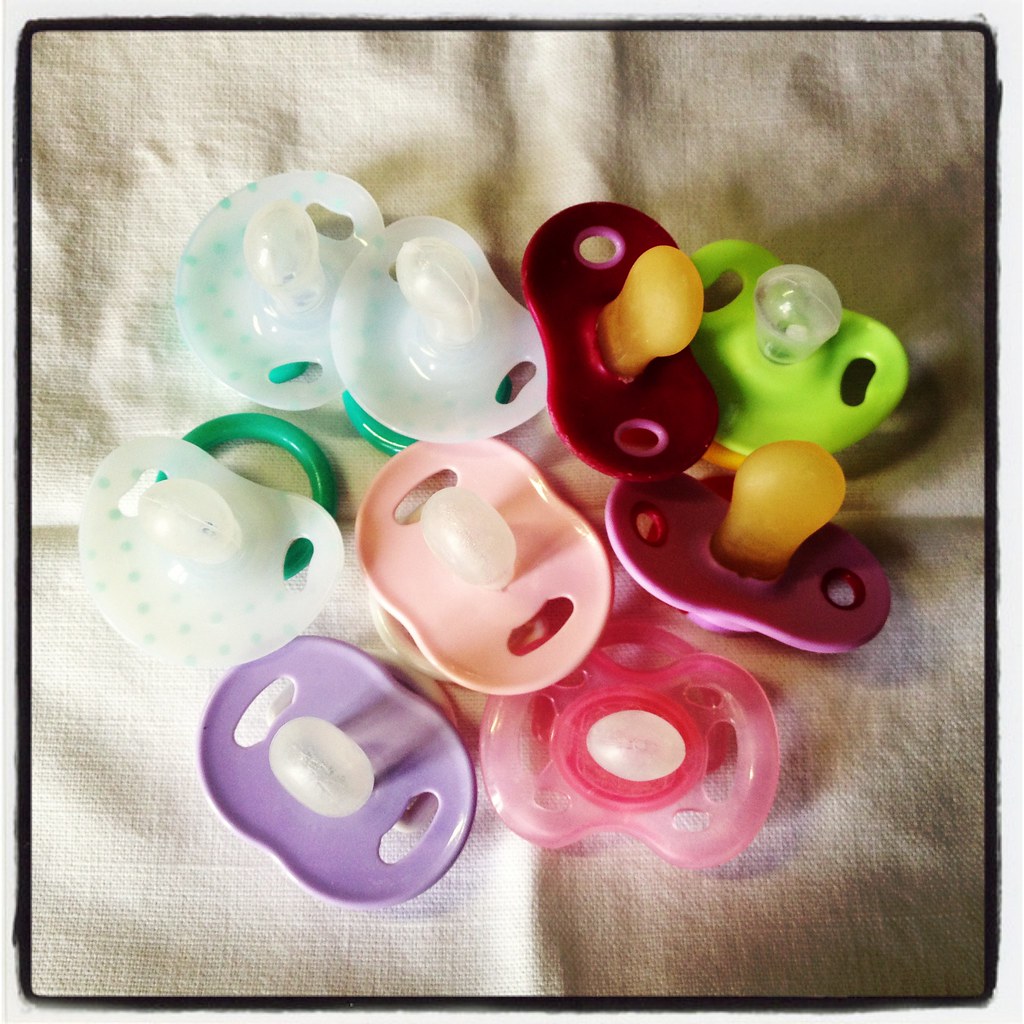In this image, a variety of baby pacifiers are artfully arranged on a beige piece of fabric, which features faint folding marks. The fabric appears somewhat porous, similar to cheesecloth. Nine pacifiers, each with its own distinct design, rest in the center, forming a compact cluster. Each pacifier has a plastic end designed for the baby to suck on, all facing upwards. 

The pacifiers come in different colors and shapes: some are rounded with holes on the sides, while others have a peanut shape with openings for ventilation. Specifically, we see a range of hues including a lime green pacifier, a medium pink, a clear pink shade, burgundy, and purple. Among them, three pacifiers are clear with small green spots and green rings. There are also two maroon ones, a light pink, a brighter translucent pink, and a purple pacifier. 

The image features a black border around the edge with a white border surrounding it, framing the scene. The diversity in pacifier designs and colors adds a vibrant touch to the overall composition.